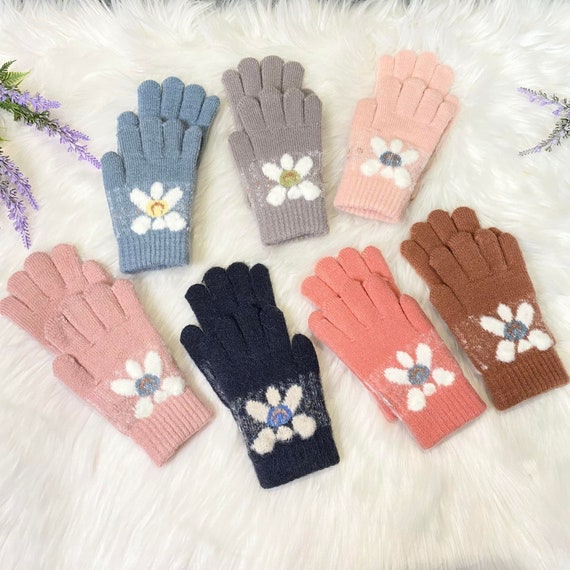This photograph showcases seven pairs of knit gloves, each uniquely colored and adorned with white flowers featuring variously colored centers. The gloves are artfully arranged on a white, fluffy surface, creating a soft and cozy backdrop. From left to right, the gloves are colored in dusty blue, hearty gray, baby pink, musty pink, dark blue, salmon pink, and rusty brown. Each glove set features an embroidered floral motif on the back of the palm, with flower centers in hues of yellow, green, blue, light brown, and tan, offering a charming burst of color. Additionally, sprigs of lavender peek out from the left and right sides, enhancing the aesthetic appeal of the composition. The gloves are laid out flat, overlapping slightly, with the fingers of each pair subtly visible, suggesting their paired nature despite their overlapping placement.